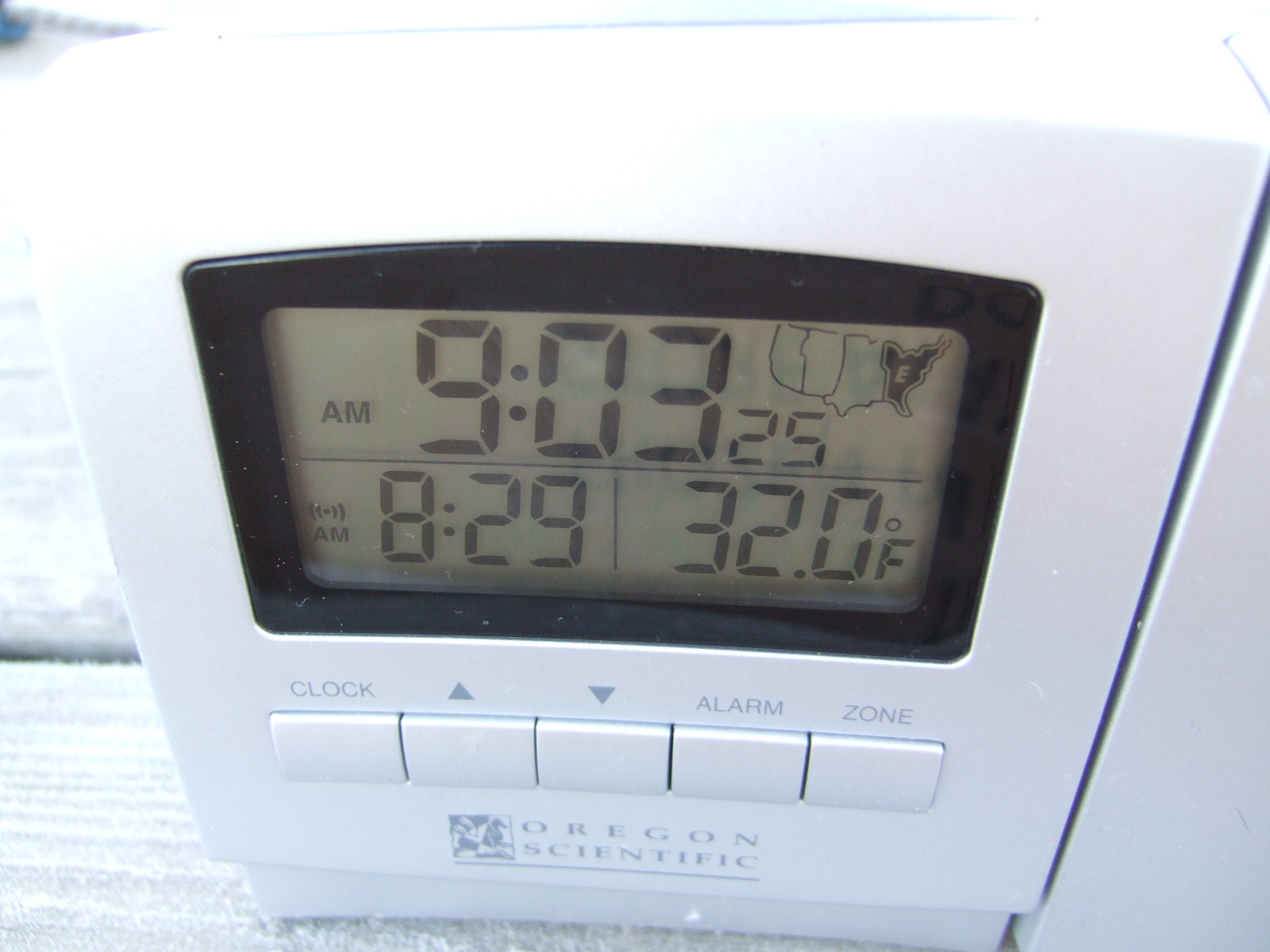This landscape-style photograph focuses entirely on a square, white thermostat. The centerpiece of the device is a smaller, rectangular, black-outlined LED screen, which displays information on a dull greenish-gray background. At the top of the screen, the time is shown in black font, reading "AM 9:03:25." Below the time, icons representing four provinces are displayed, with the far-right one filled in black and labeled with the letter "E" in white.

A thin black line separates the time display from additional information below. Underneath this line, the screen shows the previous time as "AM 8:29" in black font, followed by a vertical line and "32.0°F," indicating the temperature in Fahrenheit.

Outside the black rectangle and beneath the screen are five small, rectangular push buttons. The button on the far left, labeled "Clock," is gray, followed by a button marked with an upward arrow, another with a downward arrow, a button labeled "Alarm," and the final button labeled "Zone." Centered below these buttons, in gray text, are the words "Oregon Scientific."